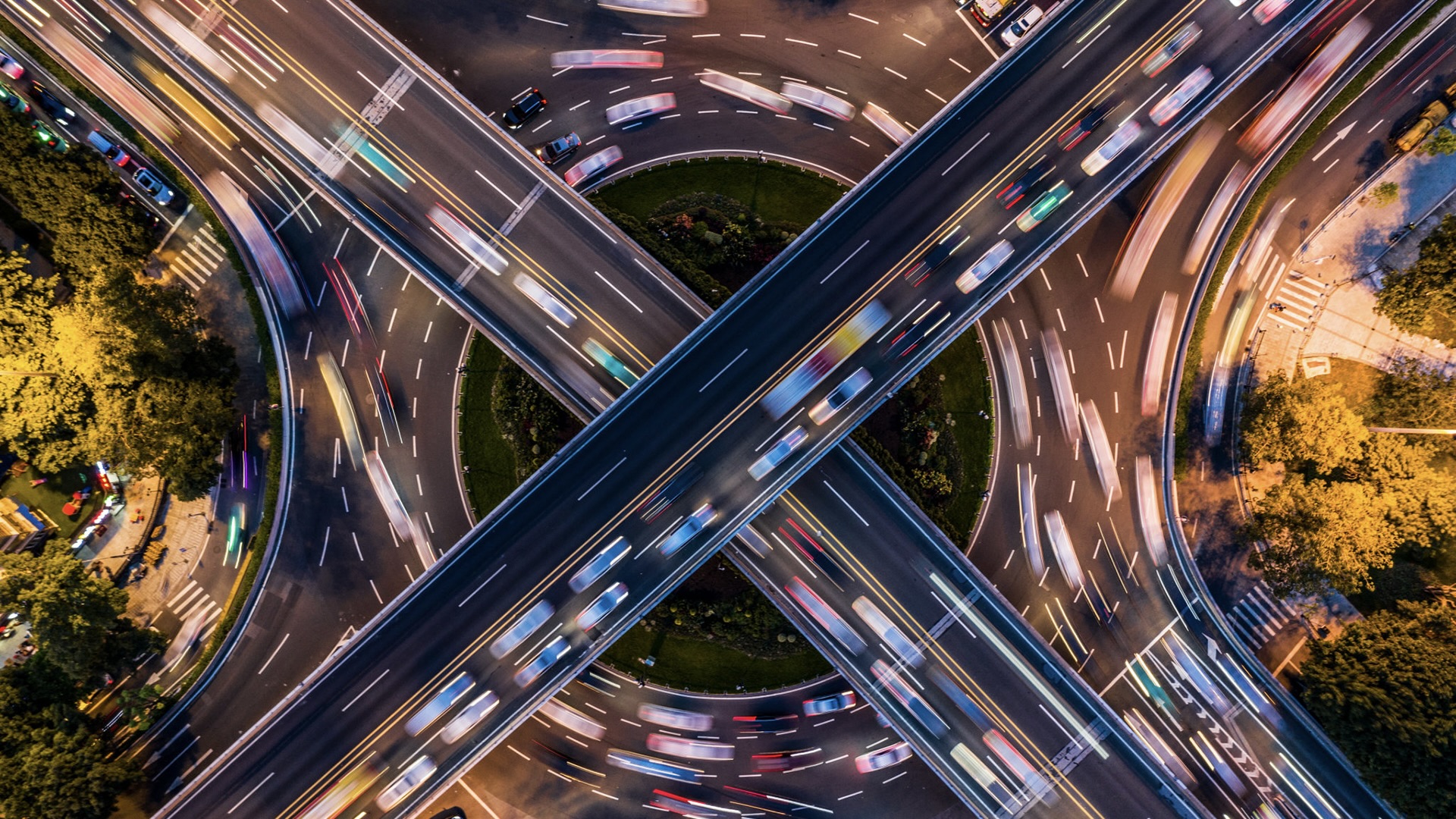This is an overhead color photograph captured from a high altitude, showcasing a complex and bustling highway interchange. The image vividly displays a massive intersection where multiple freeways and highways converge. The main visual elements include two major highways crossing each other, almost forming an X shape, with each highway comprising two lanes marked by white stripes and separated by a central double yellow line.

Below the intersecting highways, there is a large roundabout with multiple lanes, also marked by white dotted lines, accommodating traffic from at least four different directions. The photograph employs a long exposure technique, resulting in the moving cars appearing as streaks of color, giving a sense of dynamic motion and congestion. Additional roads can be seen entering and exiting the interchange, contributing to its complexity.

Surrounding the intricate web of asphalt are patches of green with trees, hinting at a few residential houses visible in the vicinity. On the periphery, sidewalks, parking lots, and crosswalks add to the detailed landscape, illustrating the intricate blend of infrastructure and urban surroundings. The meticulous layout and sheer volume of vehicles underscore the area's status as a critical junction in the highway system.